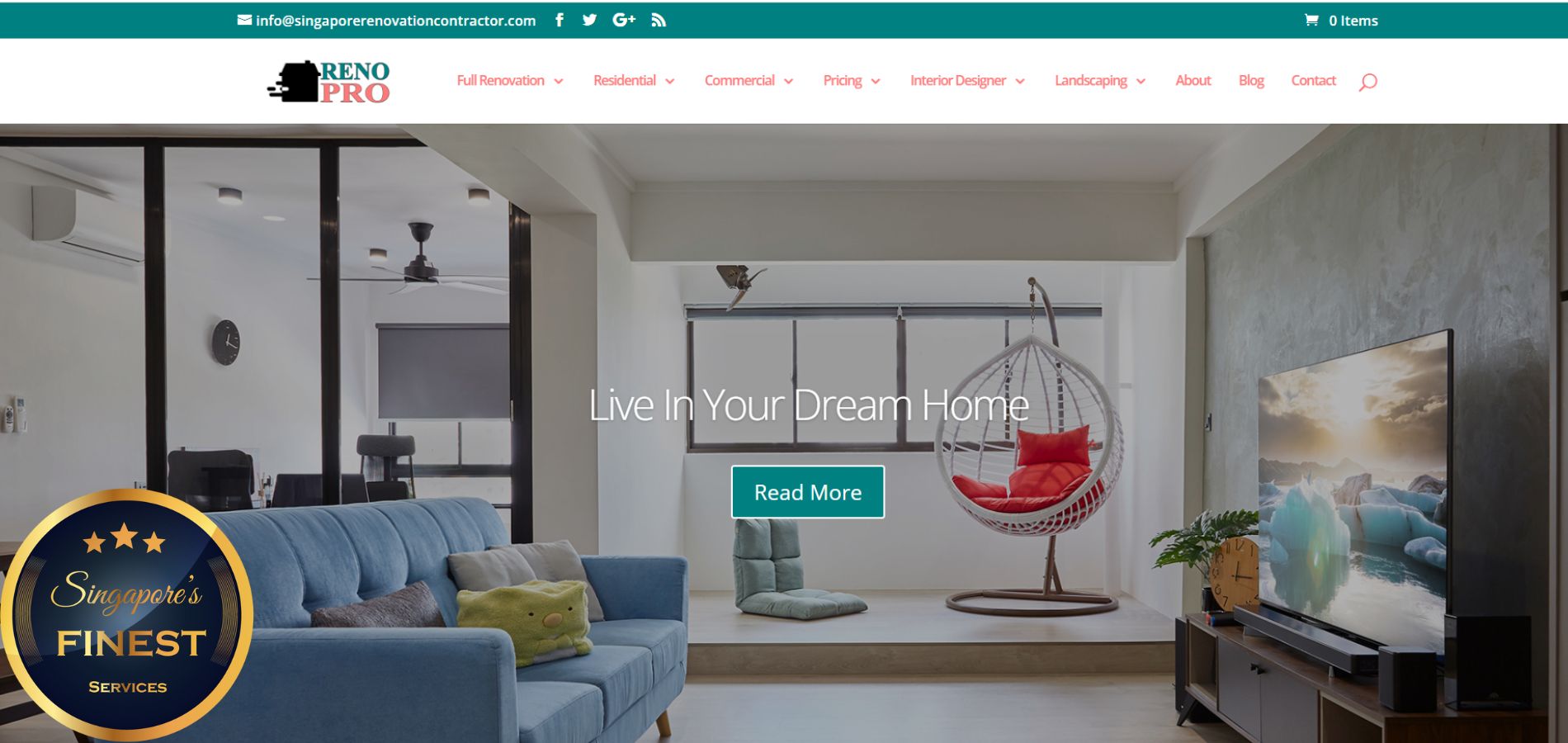This is a detailed caption for an image of a website screenshot:

The screenshot captures a website's layout prominently featuring a photograph of a stylish living space. At the very top of the page, a thin, turquoise green bar stretches horizontally from left to right. On the left side of this bar, there is an email address followed by icons for Facebook, Twitter, Google+, and Wi-Fi. To the far right, there is a shopping cart icon with the text "0 items".

Below this top bar, a white navigation bar spans across the page. On the left side of the navigation bar, it reads "Reno Pro" or possibly "Renault Pro" accompanied by a logo image. In very small red print next to the logo, illegible text is present, seemingly starting with "full". The navigation options include: Full ... (indecipherable), Something Commercial, Pricing, Interior Designer, Landscaping, About, Blog, and Contact. Additionally, there is a search option towards the right.

The main body of the webpage showcases a photograph depicting an inviting living space. To the left, a blue couch is partially visible. On the right side of the image, there is a television perched on a unit. Positioned centrally in the image, there is a hanging woven chair with vibrant red cushions. Superimposed over the photograph, white text reads "Live in your dream home" with a turquoise button beneath it that says "Read more" in white lettering, centered in the frame.

In the far bottom-left corner of the photograph, there is an emblem featuring a gold circle encasing a navy circle. At the top of the navy circle, three gold stars are visible. The interior of the circle bears the text "Singapore's Finest Services".